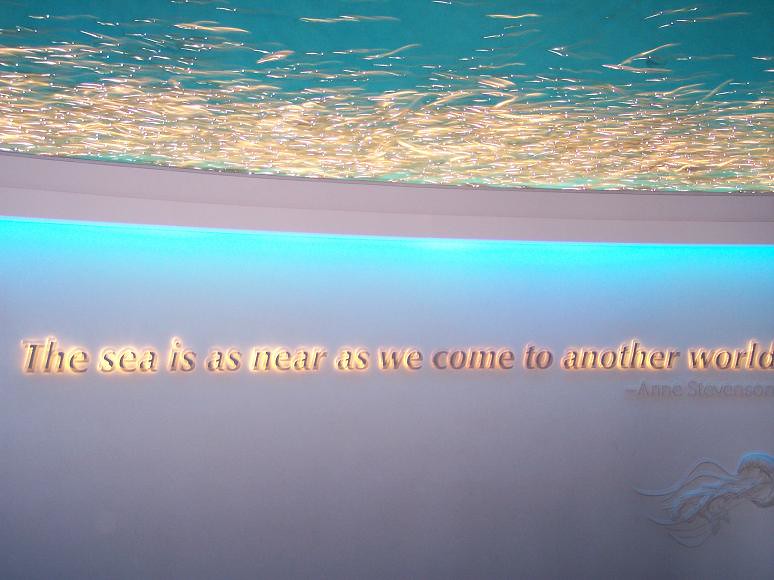The image depicts an exhibit featuring a prominent quote from Anne Stevenson, "The sea is as near as we come to another world," illuminated by lighting that highlights the text with a gold glow. Above the quote, the ceiling showcases a superimposed image of the sea, complete with flowing water and marine life such as fish, set against a bluish-green backdrop. Below the quote, the wall features embossed elements that resemble sea creatures, potentially seaweed, jellyfish, or sea crabs. A white border with blue lighting beneath it enhances the visual appeal, adding to the underwater ambiance.